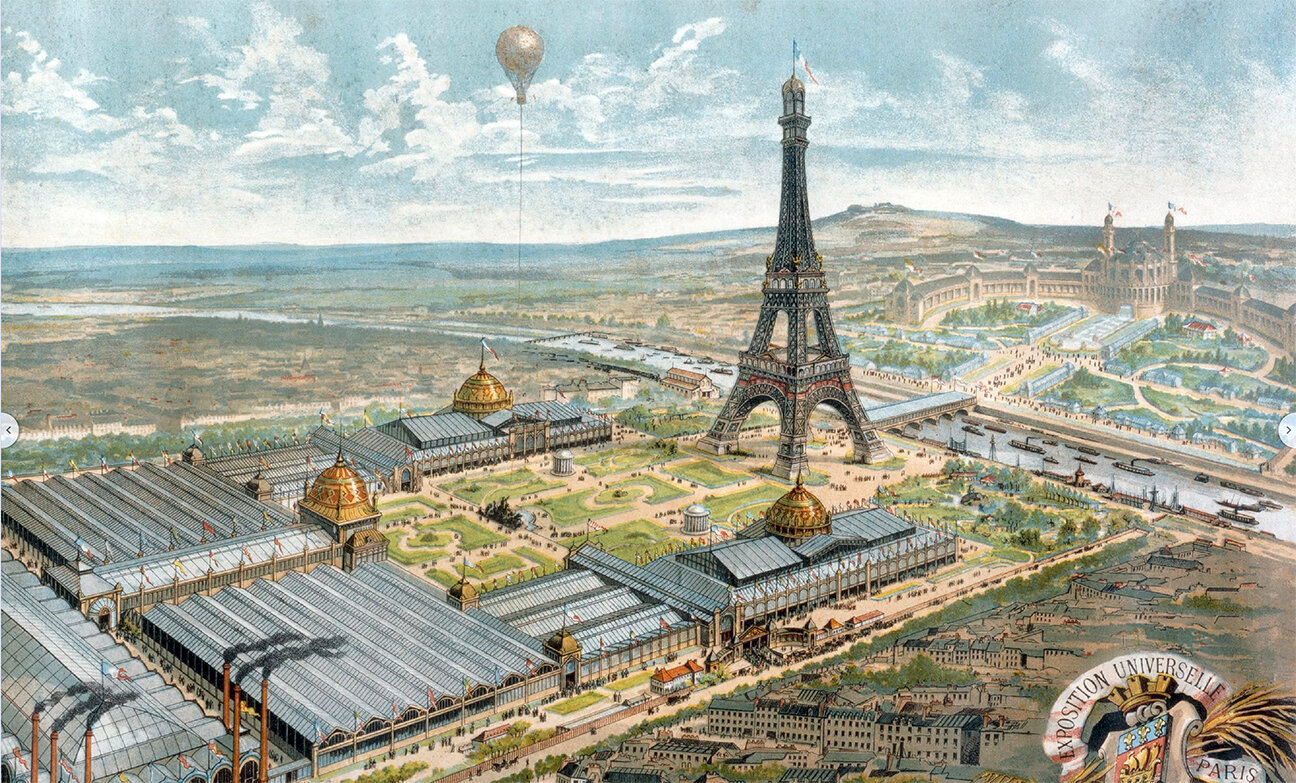This image is a detailed, full-color illustration of Paris set outdoors during the daytime, illuminated by natural light. The image is square and borderless, resembling a historical drawing or poster, and is taken from an elevated perspective. The sky occupies the upper portion, exhibiting a blend of light blue hues and feathery white clouds. Prominently placed near the upper center is the Eiffel Tower, flanked by a collection of buildings with characteristic silver and gold domes. To the upper left, a gray hot air balloon floats gracefully.

On the right, a slight hill melds into the horizon, leading to a castle that likely dates back to the French monarchy. Below the castle, a river winds its way across the scene, curving from the upper left towards the lower right. This waterway is speckled with numerous boats and intersected by a bridge. The land beside the river is densely populated with an assortment of buildings, reflecting the architectural heritage of the city.

In the lower right-hand corner, the image bears an emblem that reads "Exposition Universelle Paris," hinting at the historical and celebratory nature of the illustration. The scene captures a meticulously maintained and decorated snapshot of Paris, reflecting its iconic landmarks and vibrant urban landscape.